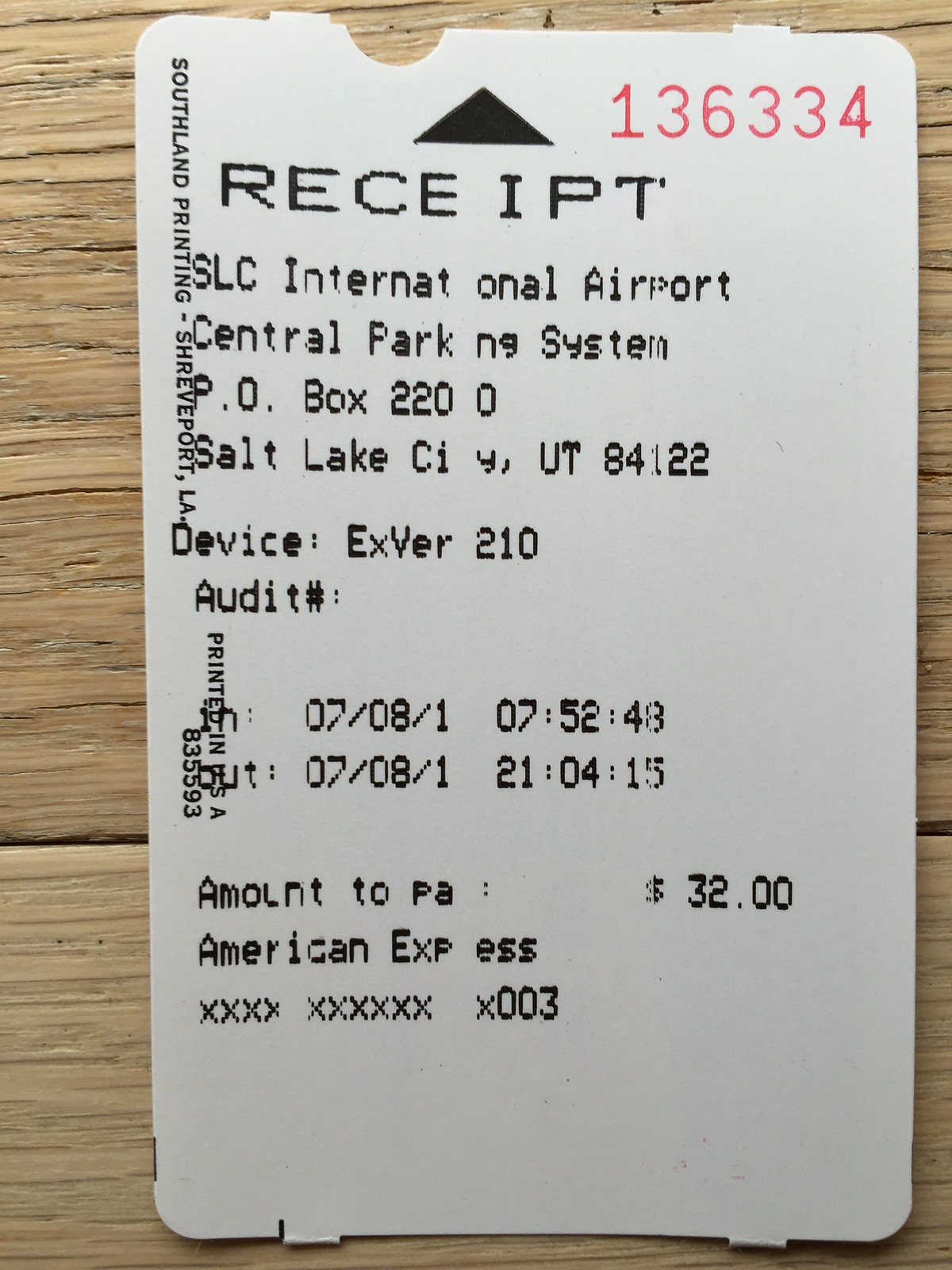A receipt, positioned vertically, lies on a rustic wooden table that features a pale light brown hue with horizontal black grains. The issued receipt, with a white background and predominantly black text, stands out due to its distinctive red print of the number "136334" located at the upper right corner. 

On the left side of the receipt, there are the words "Southland Printing, Shreveport, Louisiana," followed by "Printed in USA" and the numerical code "83559300." The top of the receipt displays a small black triangle, beneath which the word "RECEIPT" is prominently printed.

The details continue with "SLC International Airport" and the partially unclear "Central Park NG System," followed by the address "P.O. Box 2200, Salt Lake City, UT 84122." Further down, the receipt references the device identifier "EXVER210" and an "Audit Number," although the number itself is not provided.

The date and time of the transaction are next, marked as "07/08/1" at "07:52:48" for entry, and "07/08/1" at "21:04:15" for exit. Below these specifics, the receipt indicates the amount payable as "$32," charged via American Express, though the card number is partially obscured, showing as "XXXX XXXXXX X0030" with the letter "R" missing from the word "CARD."

This meticulously detailed scene captures not only the content of the receipt but also the texture and appearance of the wooden table surface beneath it, illuminating the nuanced interplay of everyday objects.